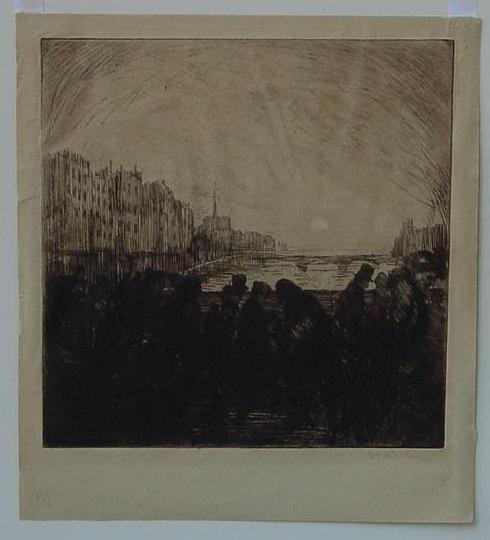The artwork is a detailed black and white ink and graphite painting, capturing a cityscape by a body of water, either a canal or a river. The scene is somewhat dark and melancholic, reflecting a grayish, overcast sky. In the foreground, a bridge teeming with silhouetted figures, many wearing hats, spans the water. Some figures move to the left while others head to the right, their detailed features obscured by the dark tones of the painting. The water beneath the bridge exhibits subtle ripples and creases, adding texture and depth. In the background, a second bridge with visible pillars extends across the water, though no people are visible on it. On the left side of the scene, a series of dilapidated buildings with cracked facades and missing corners stretch towards the horizon, leading to the vanishing point where the sun appears to rise faintly, casting minimal light. The entire scene has a scratchy, Polaroid-like aesthetic, framed on all sides with the bottom edge being slightly larger, emphasizing the painting's vintage feel. The canvas itself is rendered in a very off-white shade, adding to the artwork's evocative and somber tone.